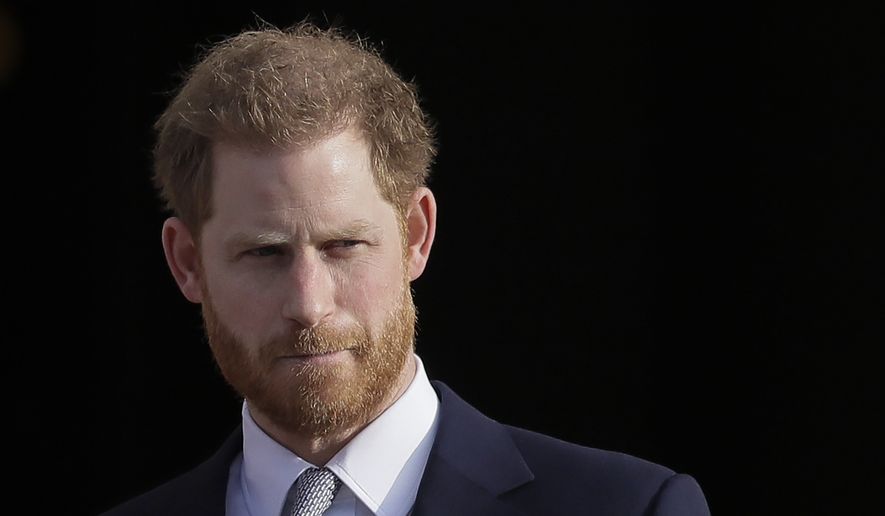This photograph features Prince Harry against a black backdrop. He has his signature close-cropped red hair with a slight balding spot at the front, red eyebrows, and a neatly trimmed red beard and mustache. His pale complexion is marked by some ruddy patches on his cheeks, nose, forehead, and around his ears. Prince Harry's hairstyle tapers into a rounded V-shape at the center with the sides layered differently from the top. He's dressed in a meticulously tailored black tuxedo paired with a white dress shirt and a patterned gray and blue tie. His ears are short and rounded, lying close to his head. Harry appears to be looking slightly downward and leering to his right, squinting as if the sun is in his eyes, revealing two frown lines between his eyebrows. His facial expression is serious, and his eyes, difficult to discern in color, reflect a contemplative mood. His attire and grooming reflect a formal, well-groomed appearance under subtle natural lighting.